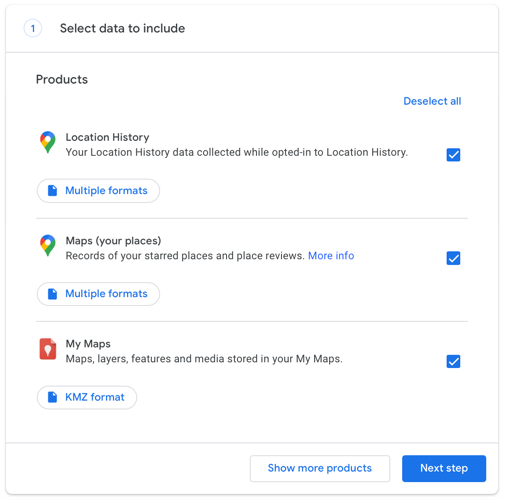The image is a screenshot of a specific section of a website interface. At the top of the page, the phrase "Select Data to Include" is prominently displayed in black text, accompanied by a blue number "1" to its left. A thin gray line runs horizontally across the page, acting as a divider.

Below this line, there is a section titled "Products," followed by another text segment: "Location History." This section explains, "Your location history, data collected while opted into Location History." Directly beneath this, the text "Multiple formats" appears.

Further down, the section labeled "Maps (Your Places)" describes, "Records of your starred places and placed reviews," also followed by the note "Multiple formats."

Continuing lower, the "My Maps" section provides details about "Maps, layers, features, and media stored in your My Maps," with "KMZ format" highlighted in blue text.

On the right-hand side of the screenshot, there are three blue squares, each containing a checkmark. Above these squares, the text "Deselect All" is displayed in blue.

At the bottom right corner of the page, two buttons are visible: "Show More Products" in blue text on a white background, and "Next Step" in white text on a blue background. The entire interface is set against a white background.